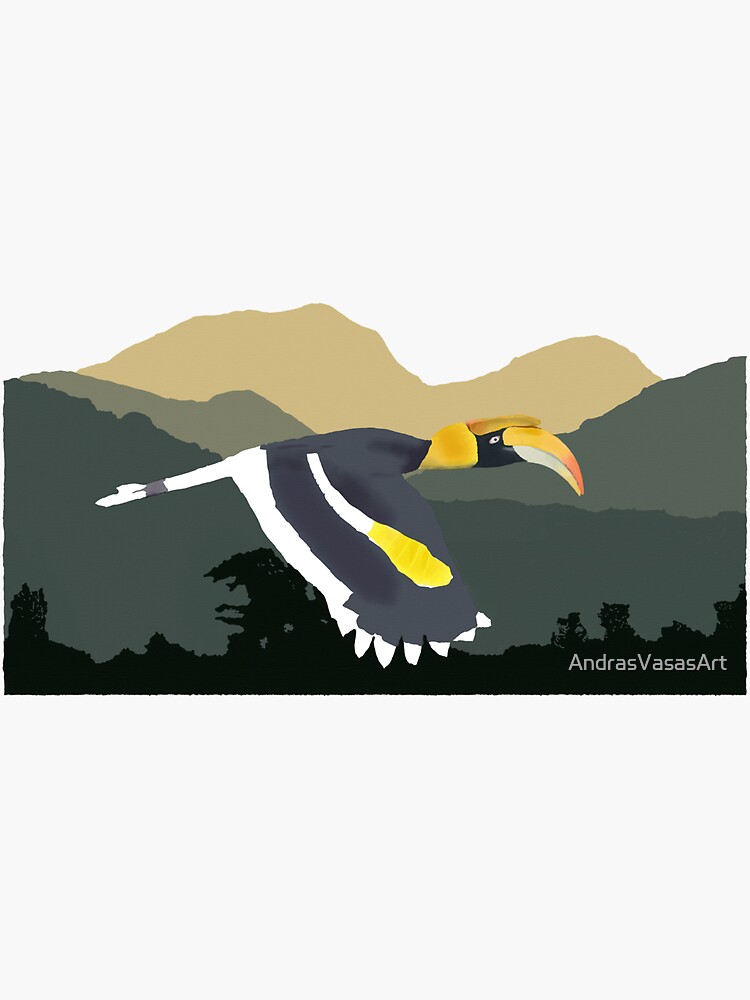This detailed description from multiple perspectives reveals a singular image of a vibrant digital artwork created by Andras Vasas Arts, depicting a majestic Great Hornbill. The bird, featured in this watercolor-inspired abstract piece, showcases striking color contrasts with a black upper body and a white lower body. Its large wings are primarily black, decorated with yellow and white streaks, and the tips are stark white. A notable yellow crown adorns its head, complementing its distinctively large, yellow and red horn-like beak. The tail, small yet distinctive, is predominantly white with a subtle grey stripe. The Great Hornbill appears to be soaring gracefully over a dramatic landscape of multicolored valleys and mountains, ranging from dark green to light green and orange-brown hues. The sky in the background is depicted in plain white, emphasizing the bird's striking features and the scenic, tiered canyon-like valleys below. The artwork is signed by "Andras Vasas Arts" in the bottom right corner, affirming its creative origin.